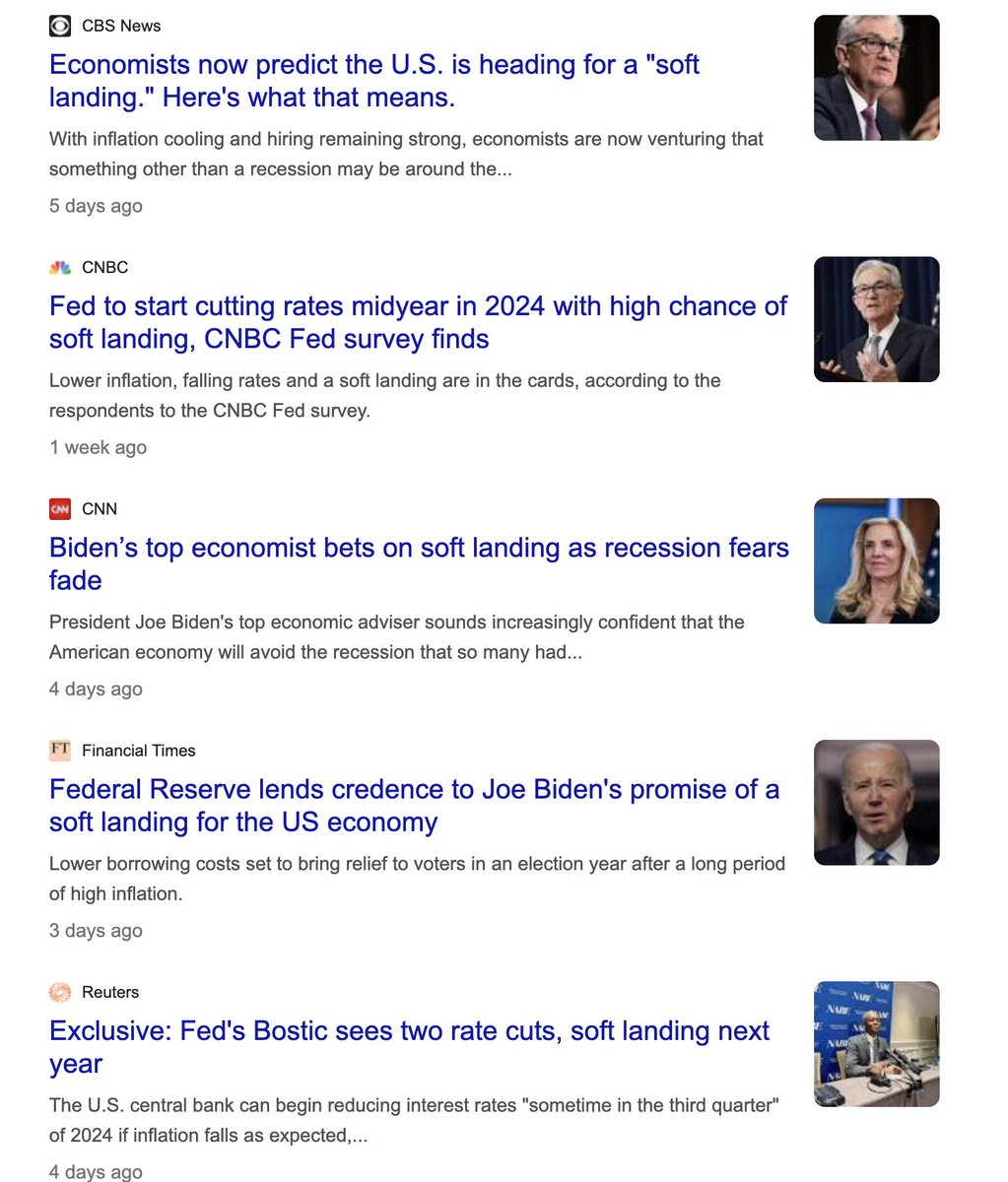This infographic features a white background and is segmented by various prominent news logos each highlighting recent economic predictions:

1. **CBS News**: Positioned at the top with a black square featuring the iconic CBS eye symbol. The accompanying text notes that economists now predict the U.S. is heading for a "soft landing," referencing cooling inflation and strong hiring trends. This segment is dated five days ago and includes a picture on the right-hand side.

2. **CNBC**: Displayed with the colorful peacock logo, CNBC reports that the Federal Reserve is expected to start cutting rates by mid-2024, increasing the likelihood of a soft landing. The CNBC Fed Survey suggests this, with additional highlights on lower inflation and falling rates. This section is dated one week ago and includes a picture of a man.

3. **CNN**: Featured in a red box, CNN's headline states that President Biden's top economist is betting on a soft landing for the economy, with recession fears diminishing. This update, dated four days ago, is accompanied by a picture of a woman.

4. **Financial Times (FT)**: Marked by a pink box, the Financial Times notes that the Federal Reserve's decisions support Joe Biden's promise of a soft landing for the U.S. economy, with lower borrowing costs potentially easing voter concerns in an election year. This was reported three days ago and includes a picture of Joe Biden.

5. **Reuters**: Displayed with a red world logo, Reuters shares an exclusive report that Federal Reserve official Bostick anticipates two rate cuts next year, aligning with the prediction of a soft landing if inflation decreases as expected. This segment is dated four days ago and features a picture of a man.

Each news outlet provides a distinct perspective on the anticipated economic developments, collectively forecasting a "soft landing" rather than a recession for the U.S. economy.